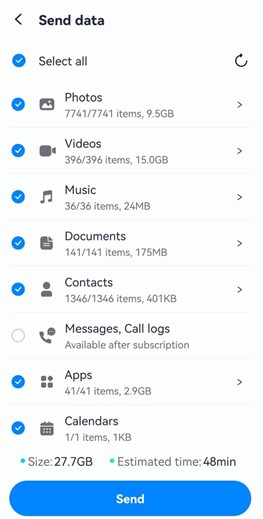### Detailed Caption:

In portrait mode, the screenshot displays a data transfer interface. The upper left corner features a "Send Data" title accompanied by a black back arrow. Below this, the interface is organized into nine rows, each containing an icon on the left and a checkmark box even further to the left.

1. **Select All**: A blue checkmark indicates that all items are selected.
2. **Photos**: Selected.
3. **Videos**: Selected.
4. **Music**: Selected.
5. **Documents**: Selected.
6. **Contacts**: Selected.
7. **Messages/Call Logs**: Grayed out and unavailable, marked "available after subscription."
8. **Apps**: 41 out of 41 items selected, totaling 2.9 GB.
9. **Calendar**: 1.1 items selected, totaling 1 KB.

At the bottom, two aqua circles display:
- **Total Size**: 27.7 GB
- **Estimated Time**: 48 minutes

A notable feature of the interface is a large blue button situated at the very bottom, which, despite the importance of its function, is marked by very small text that reads "Send". The button is disproportionately blank, with ample unused space.

Overall, the screenshot captures a user interface preparing for data transfer, with all categories except for messages/call logs selected, projecting a transfer duration of approximately 48 minutes.